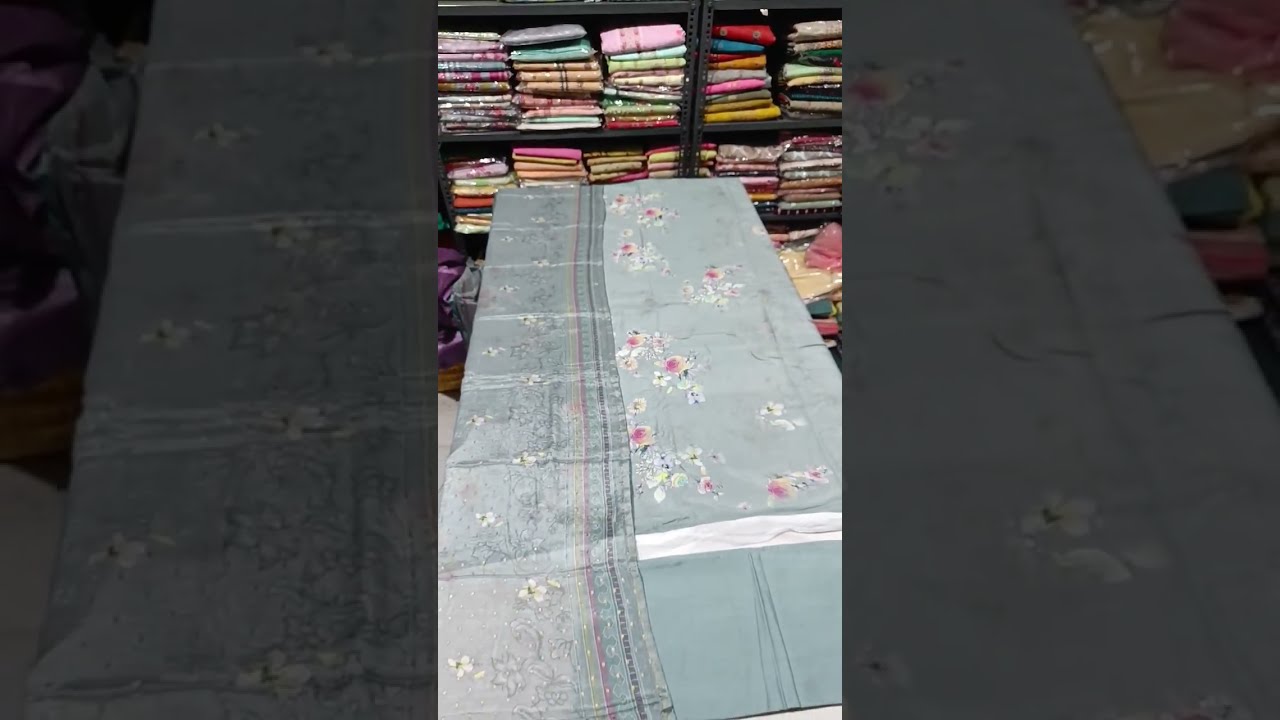This photograph depicts a neatly arranged fabric store. In the foreground, a table is draped with a striking blue tablecloth adorned with pink and white floral patterns and stripes. This focal point hints that the store specializes in textiles rather than ready-made clothing. The background reveals a set of metal shelves, painted dark gray, which hold multiple neatly folded pieces of cloth in vibrant colors—purple, pink, turquoise, blue, white, red, orange, yellow, and more. These cloths are arranged in reams and stacks, suggesting a well-organized space catering to sewing and embroidery enthusiasts. The overall scene suggests a quiet moment in a store designed for customers looking to purchase textiles for various creative projects.